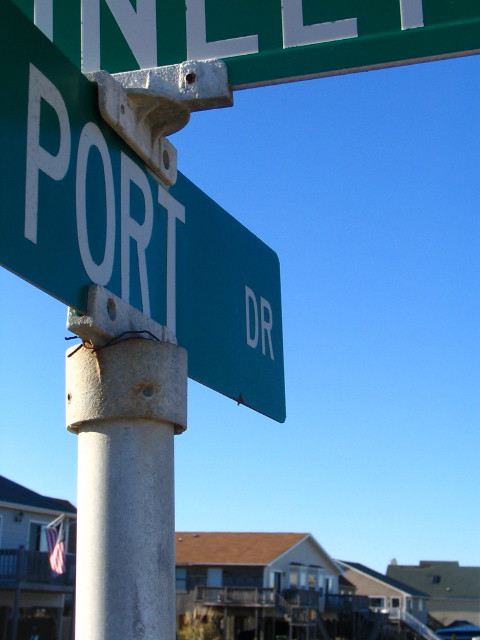The image features a street sign prominently displaying "Port Drive," mounted on a silver metal pole. The pole shows signs of weathering, with rust visible around some of the screws. At the top of the pole, a small red object resembling a tie or string is attached. Above the "Port Drive" sign, another street sign partially protrudes with visible letters "N" and "LL," although the full name is obscured.

In the background, there are several houses that evoke a coastal vibe. These homes are elevated with decks on their second levels, hinting at a possible view of the ocean. The lack of tall trees further suggests a beachfront location. The overall scenery conveys a tranquil, seaside neighborhood atmosphere.